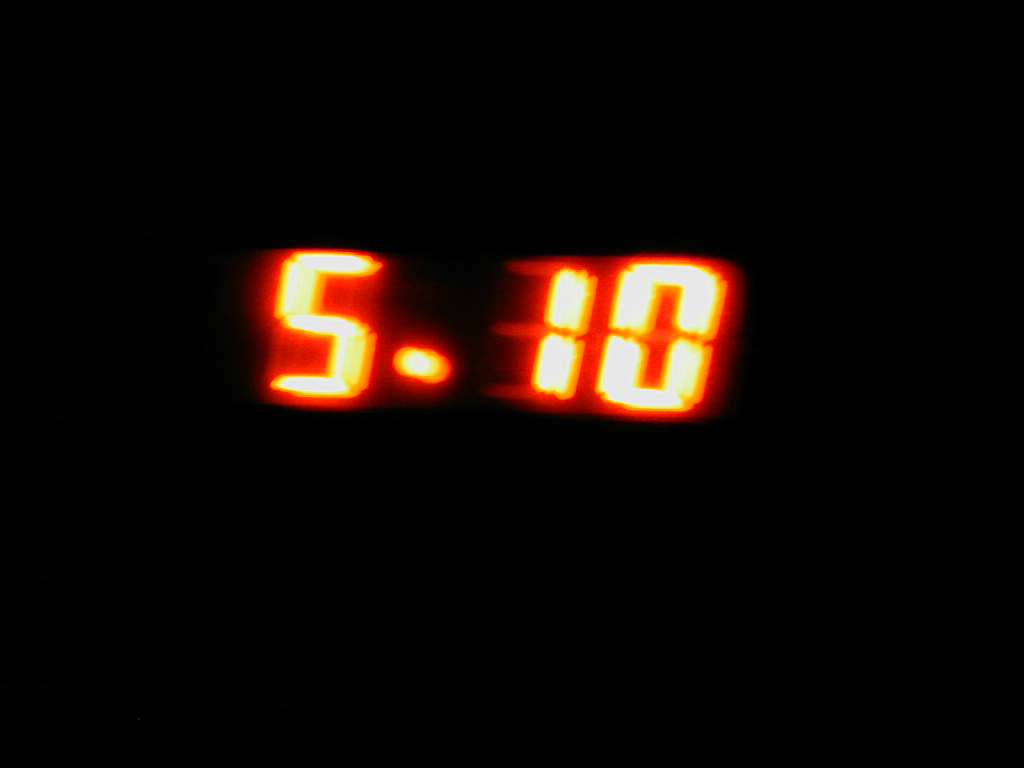In this image, a pitch-black background starkly contrasts with the luminous display of a digital clock. At the center of the image are the glowing numbers "5.10," displayed in a digital font. The numbers are brilliantly illuminated in vibrant shades of white and yellow, complemented by an outer glow in a reddish-orange hue. The composition of the numbers is precise: the "5" is formed by five rectangular segments, the dot is a simple, glowing point, the "1" comprises two rectangles, and the "0" consists of six rectangles forming two U-shapes with a gap in between. The overall effect is dynamic, with a slight blur suggesting motion or a long exposure, intensifying the multicolored glow. This glowing effect extends outward, casting a colorful shadow that deepens the intensity of the orangish-red tones, making the digits appear both vivid and slightly reflective, as if lit from within.